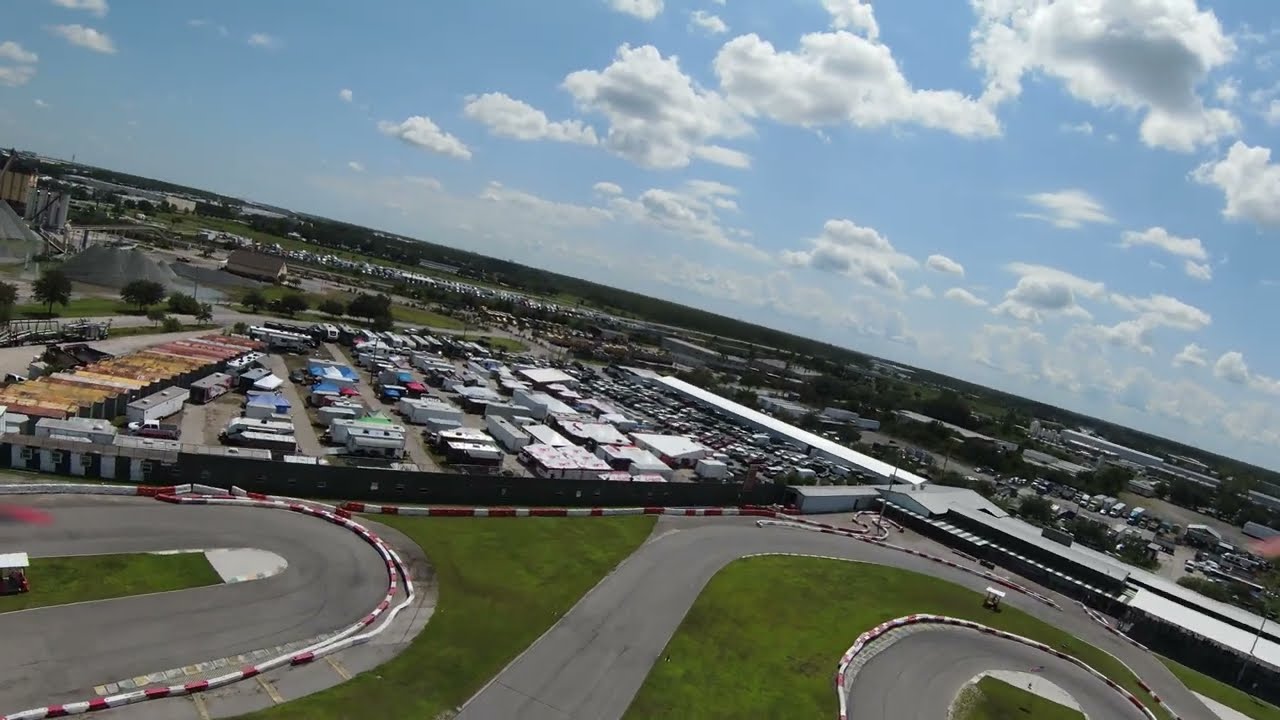An aerial view of an industrial complex during daytime, showcasing a detailed layout beneath a bright blue sky dotted with puffy white clouds. In the immediate foreground, a well-maintained green lawn is interspersed with paved strips resembling highways or driveways, featuring a distinct spiraling design with red and white barricades suggestive of a racetrack. Adjacent to this green area lies a large expanse of paved surfaces dotted with a variety of buildings including industrial plants, warehouses, factories, and commercial structures. Significant among these is a long factory-like building situated at the edge of the paved area. Scattered throughout this expanse are numerous trailers, RVs, cars, trucks, and buses parked in designated areas, indicating a bustling environment. Behind a black fence bordering the racetrack, more buildings and a parking lot can be seen, surrounded by trees and further interspersed with structures extending towards the horizon. In the distance, an industrial plant with a mound of gray sand or dirt transitions into a flat landscape dotted with trees, underlining the area's mixed-use nature. No people are visible in this expansive and diverse scene.